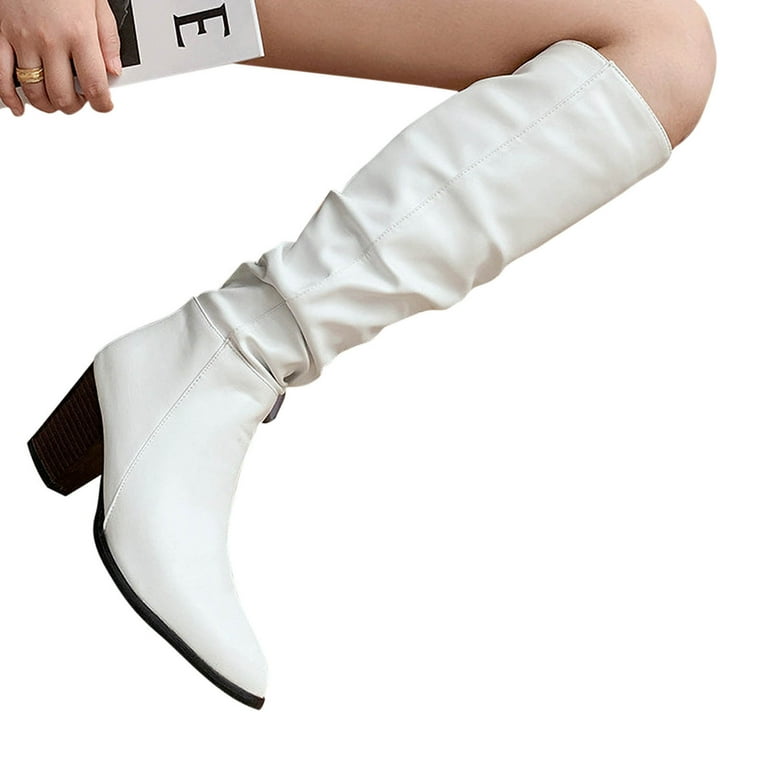This detailed close-up photograph, captured in an advertisement style, showcases a white woman's leg partially clad in a knee-high, slouchy, white leather boot. The boot, characterized by creases running down towards the ankle, features a black woodgrain heel and a black sole, alongside a pointed toe design. The leg is bent at the knee, emphasizing the boot's length and form. In the top left corner of the image, the woman's hand, adorned with a gold ring on her ring finger, holds a white and black booklet prominently displaying a large black letter "E". The background of the photograph is white, highlighting the contrast and details of the boot and the booklet.